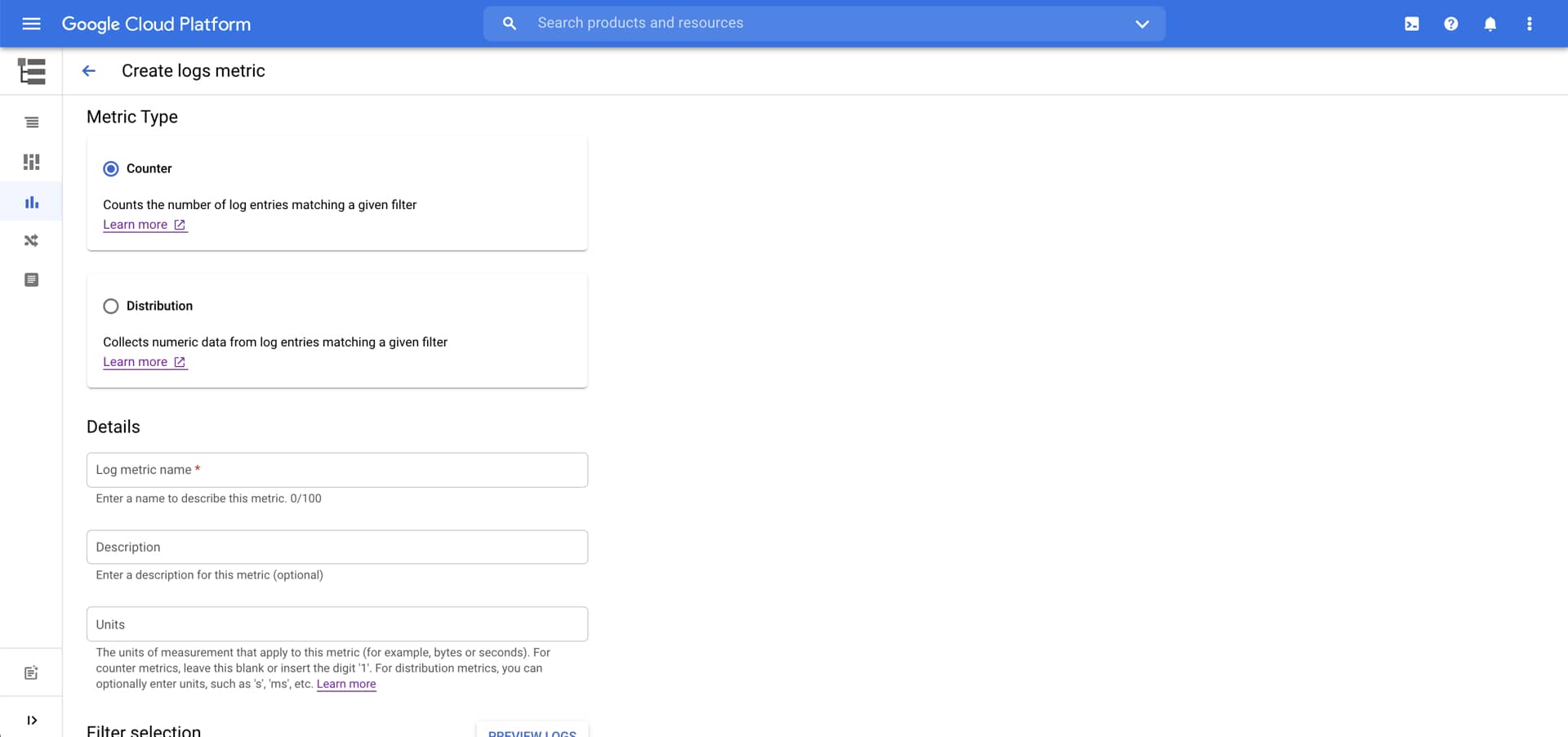This screenshot displays a section of the Google Cloud Platform interface. 

At the top of the interface, a blue header features "Google Cloud Platform" on the left. Positioned to the right is a search bar with placeholder text that reads "Search products and resources" in white. Adjacent to the search bar is a pull-down arrow. Further to the right are three icons: a question mark within a white circle, a notification bell, and a three-dot menu icon.

The main section below the header has a white background and is titled "Create Logs Metric." To the left of this title is a blue arrow. Under the title, there is an option for "Metric Type," represented by a blue-filled circle labeled "Counter," which is defined as counting the number of log entries that match a given filter. Accompanying this is a purple underlined link labeled "Learn More."

A horizontal gray line separates the next section, which is titled "Distribution" in bold black text. This section describes the collection of numeric data from log entries that match a given filter, with another "Learn More" link included.

Towards the bottom, a section titled "Details" in bold black text features a search bar prompting the user to "Log Metric Name," where one can enter a name to describe the metric being created.